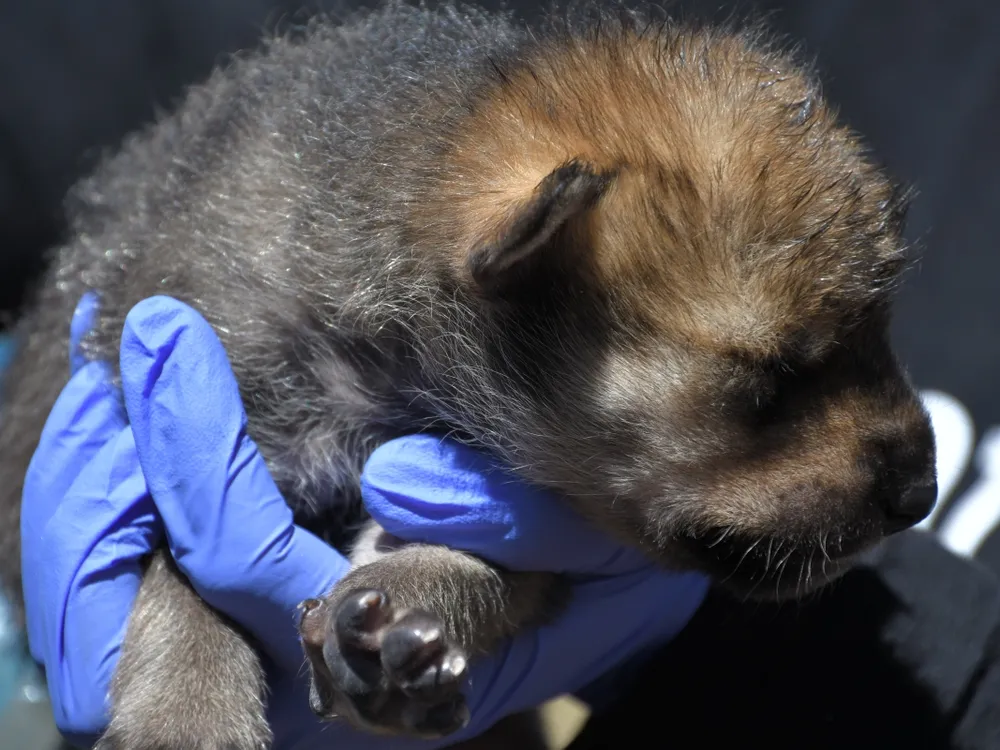In this close-up image, a tiny, very young puppy, likely just a few days to a week old, is cradled in a gloved hand. The background is completely black, making the tender scene in the foreground the focal point. The person holding the puppy wears blue sterile gloves, hinting at a veterinary setting. The puppy's eyes are closed, indicating it is either a newborn or asleep, and its delicate frame is characterized by a coat of dark black and gray fur with patches of brown. The puppy's small paws and black foot pads add to its fragile appearance. Only a few fingers of the hand are visible, suggesting a careful and gentle grip, typical of someone providing medical care or nurturing a young animal in need.